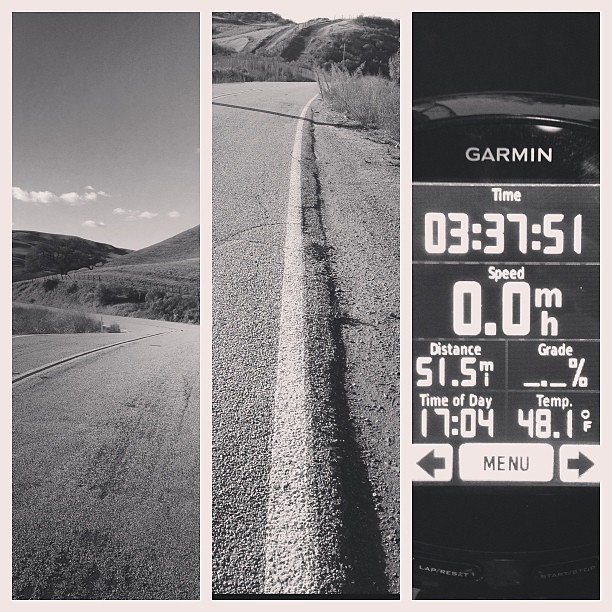The image consists of three vertically aligned, black-and-white photographs within a light gray or off-white border, each occupying one-third of the space. The first photo on the left captures an open field with a winding road stretching towards distant rolling hills, set under a mostly clear sky with a few fluffy clouds. A tree, a fence, and scattered grass are visible, contributing to the picturesque hilly countryside. The middle photograph zooms in on a paved road's edge, highlighting the white line that demarcates the boundary, with scrub grass growing tall beside it and small hills and a fence in the backdrop. The photo on the right is a close-up of a Garmin device screen, displaying detailed metrics: a time of 3 hours, 37 minutes, and 51 seconds, a speed of 0.0 mph, a distance of 51.5 miles, a grade of 0%, a time of day reading 17:04, and a temperature of 48.1°F. The interface includes buttons for navigation, a menu, and options to lap reset and start/stop.